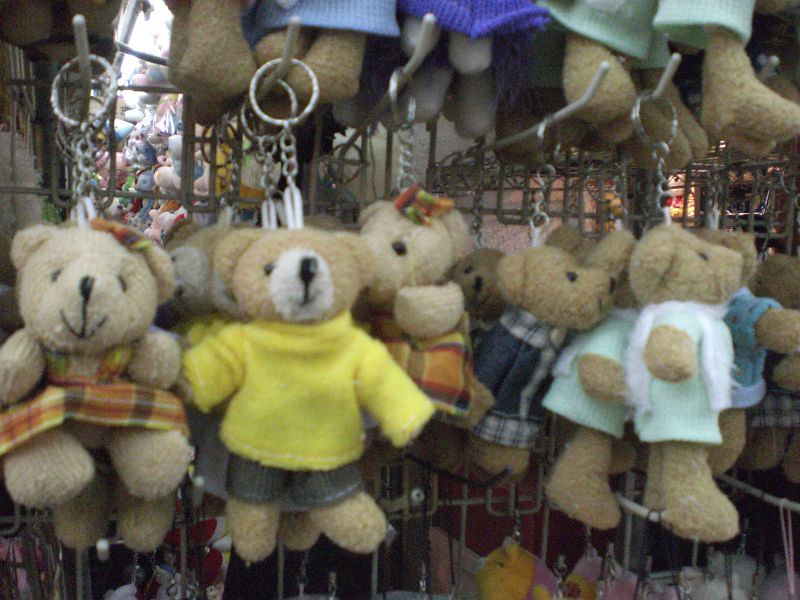This photograph depicts a street vendor's stall, possibly at an outdoor market or circus, showcasing an array of light brown teddy bear keychains. The teddy bears are adorned in various outfits and are arranged in a horizontal line, attached to a series of five metal hooks on a vertically striped metal wall. Starting from the left, the first bear is dressed in a checkered flannel shirt with red, yellow, and black colors, accentuated by a small flower on its head, indicating it might be a female bear. Next to it, a bear wearing a yellow sweater and gray pants is missing its right eye, giving it a unique characteristic. The third bear mirrors the first, with a similar checkered dress and a bow tie. Moving further right, the fourth teddy wears a dark blue plaid jacket. Finally, the last bear in the row sports a light green or teal sweater. The detailed clothing, such as shirts, pants, jumpers, and sweaters, provides each teddy bear with a distinct personality. Behind these prominently displayed bears, additional stuffed animals or merchandise can be seen, hinting at the vendor's extensive collection.